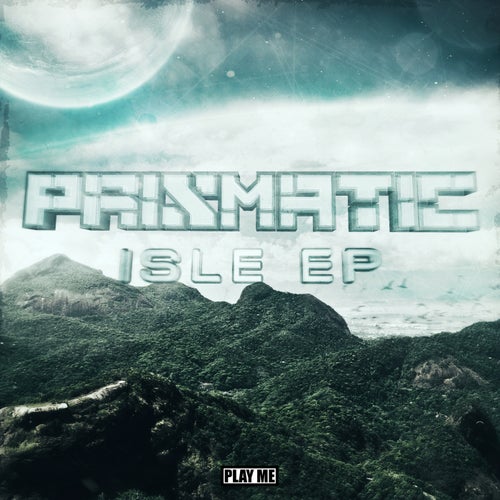The image in question appears to be a slightly blurry cover, potentially for a video game or an EP album. Dominating the upper part of the cover is a sky that blends dark blue and white hues, giving it a cosmic or outer space skyscape feel. In the upper left-hand corner, there is an outline of a white moon among the clouds. Central to the image, bold block letters spell out "PRISMATIC" in a semi-transparent font allowing the sky to show through. Immediately below, in a thinner font, the words "ISLE E.P." are displayed. The lower portion of the image features dark brown and gray rocky mountains or hills, with some birds flying toward the middle right side, adding a sense of motion. At the very bottom, a white rectangle contains the text “PLAY ME” in black, likely inviting the viewer to engage with the content, whether it be a game or music.